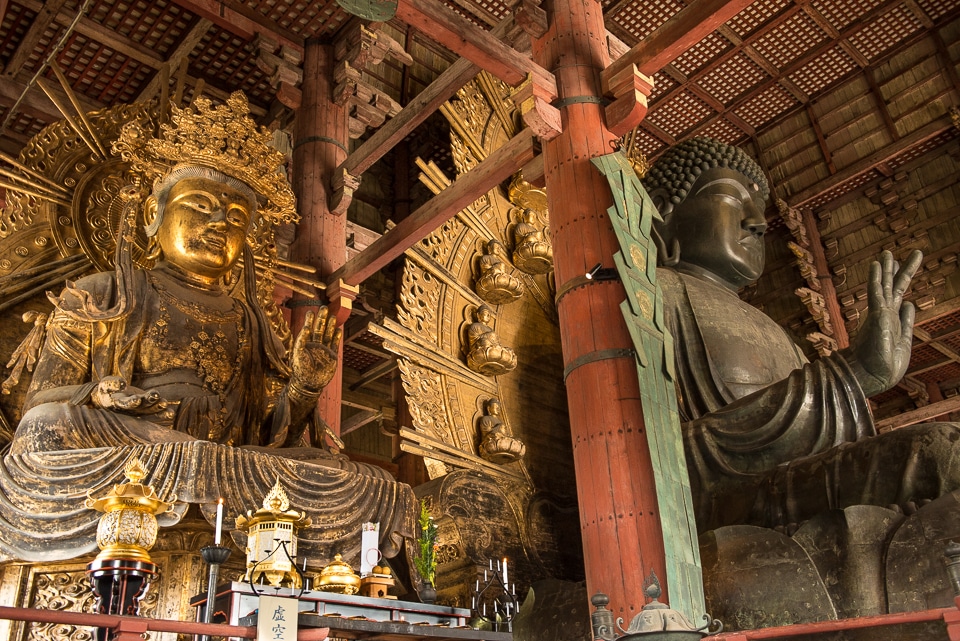This color photograph depicts the interior of an East Asian temple, showcasing rich architectural and cultural elements. Dominating the scene are two large seated statues that convey a sense of ancient reverence. The statue on the left is golden, adorned with a gold crown and intricate gold robes, its left hand raised with the palm open, reminiscent of classic Indian style poses. To the right, partially obscured by a large wooden pillar, is a statue of a Buddha-like figure with stylized curly hair, its right hand extended upwards. This statue, with a dated, slightly green patina, appears to be made of copper or bronze. Both statues are nearly as tall as the red wooden pillars that support the temple's wooden ceiling. In the foreground, traditional gold incense containers are neatly arranged on a table, enhancing the sacred ambiance of the space. The intricate support beams of the ceiling add to the grandeur of this interior, emphasizing the timelessness of the architecture.